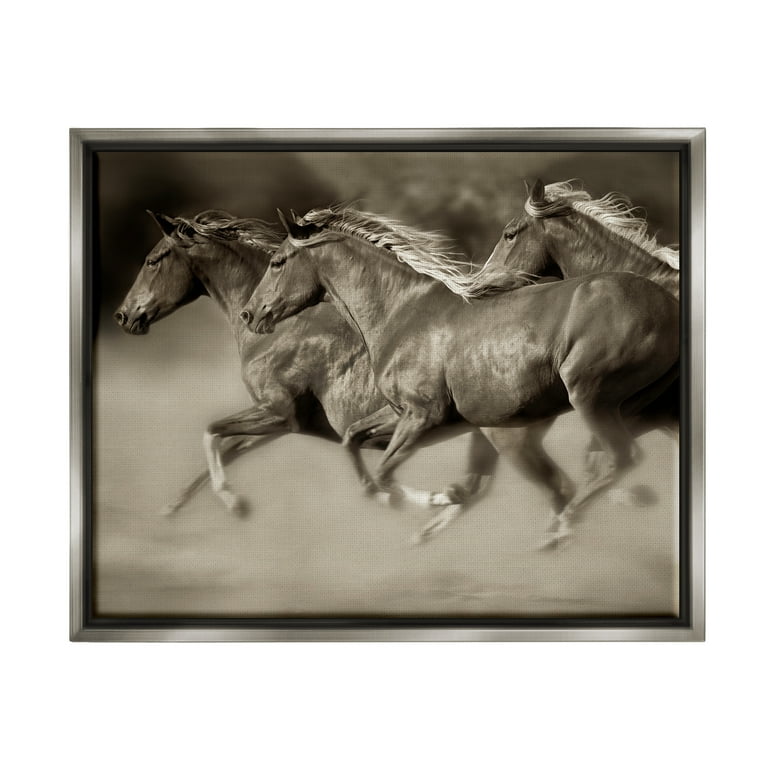In this sepia-toned portrait, three light-colored horses are captured in mid-gallop, their hooves seemingly suspended in the air as they run at high speed towards the left over a sandy terrain. The composition is predominantly in shades of brown, giving it a dark, monochromatic feel. The horses are positioned in a line, closely grouped together, accentuating their matching white socks on their feet. The central and right horses feature striking white manes, while the leftmost horse stands out with a darker, brown mane and a slightly richer fur coat. The background is indistinct, evoking a sense of open space, possibly a field or a barn area, which enhances the dynamic and free-spirited nature of the scene.